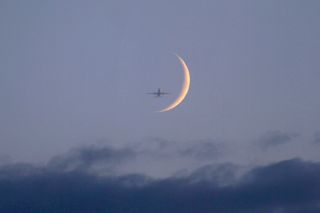This is a very small, low-resolution photo taken from the ground, looking up at the sky just before it gets completely dark. Dark grey, almost black, wispy clouds cover the bottom 20% of the image, contrasting against a lighter greyish-blue sky above. Centered in this sky is a very thin, crescent moon with a white and light yellow tint, looking almost like an eclipse. Positioned just to the left of the moon is the small silhouette of a commercial airplane, creating the impression that the plane is flying toward the viewer. The upper part of the sky is clear, giving a serene backdrop to the delicate moon and tiny aircraft.